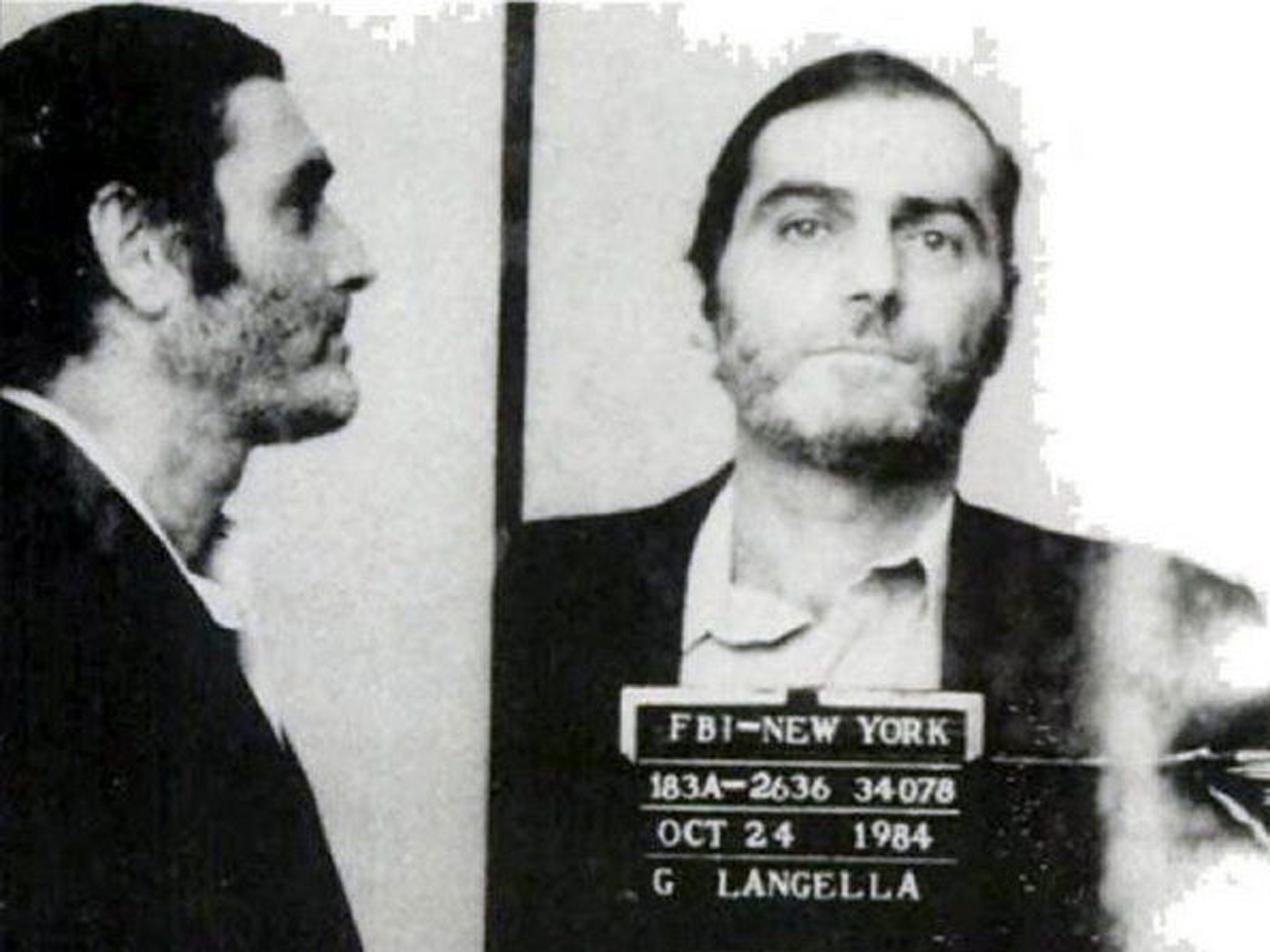This black and white mugshot features two images of a bearded male with dark, jet-black hair and sideburns; one is a side profile on the left, and the other is a frontal view on the right. He has a five o'clock shadow, and is dressed in a dark suit jacket over an unbuttoned white shirt, lacking a tie. The man is not smiling and bears a tight-lipped, grim expression. Beneath the frontal image, a sign reads "FBI New York, 183A-2636-34-078, October 24, 1984, G. Langella" in white text on a black background. This sign provides details about the arrest, including the location, date, and the individual's name.